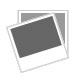The image depicts an artistic rendition of a kayaker navigating through rough, foamy whitewater. The kayaker, positioned in a single-person yellow kayak, is shown from an overhead view. He is wearing a black and red jersey with the number 67 prominently displayed on his back, along with a blue helmet and a blue and black wetsuit. The kayaker is actively paddling with a double-sided oar that features yellow blades and a black shaft. Above the scene, the text "Polo 07 Kayak Expedition" is written in white against a backdrop of turbulent blue water, signifying a competitive event. The water is depicted as intense and dynamic, partially overflowing the kayak, adding to the sense of excitement and energy in the image.